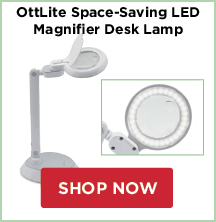The image features a clean, white background with a thin, green border outlining a square. Inside the square, bold black text reads: "Autolight Space-Saving LED Magnifier Desk Lamp." This text is centered at the top of the square, providing a clear and prominent title. On the left side of the square, there is an image of a sleek white desk lamp, showcasing its modern design. Above the lamp image, a close-up of the circular LED light is displayed, highlighting its bright and efficient illumination. At the bottom right corner, a vibrant red action button with bold white text invites viewers to "Shop Now," encouraging immediate engagement with the product.